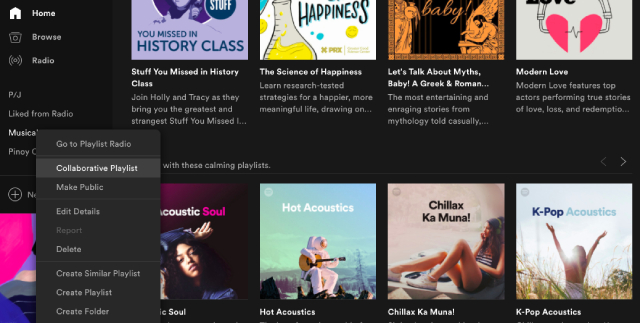The image showcases a user interface with a predominantly gray background. On the left side, there's a vertical menu bar in a darker gray with white text. The menu options, listed from top to bottom, include "Home," "Browse," "Radio," followed by a section labeled "B/J." Underneath it, there are options for "Light from Radio" and "Musical," the latter highlighted but partially obscured by a pop-up menu.

The pop-up menu for "Musical" features options like "Go to Playlist Radio" and "Collaborative Playlists," with the latter selected. The right side of the image, which occupies the majority of the space, is divided into two rows. Each row contains four blocks, each block displaying a thumbnail, a title, and a brief description. The first row includes thumbnails for "Stuff You Missed in History Class," "The Science of Happiness," "Let's Talk About Myth, Baby," and presumably additional entries following the same format, though the full list is cut off.